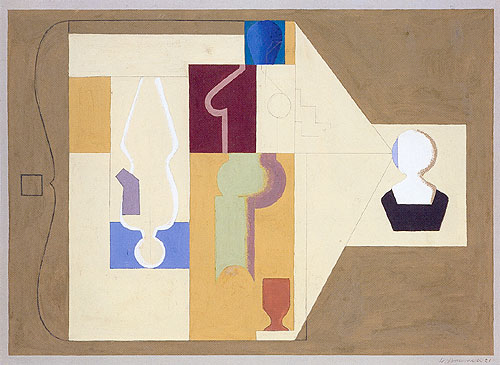This abstract oil painting on a brown background features a central shape resembling a house turned on its side, rendered in white with a triangular extension pointing right. The house shape contains numerous geometric forms, including squares and circles, with colors ranging from blue, purple, and pink to maroon, yellow, dark black, and brown. The painting's background transitions to a light cream color inside the edges. To the right, a spherical globe rests atop a hexagon or pentagon, reminiscent of a perfume bottle. The faintly rendered figure of a woman's torso, dressed in a blouse, appears on the far right. Meanwhile, the left side of the painting showcases an upside-down human figure next to a blue square and a white vase, set against a fluid interplay of beige and darker purple hues. A distinct horizontal line runs across the top, morphing into a curly brace along the left side. The intricate arrangement of obtuse forms and human elements adds depth to this enigmatic composition.